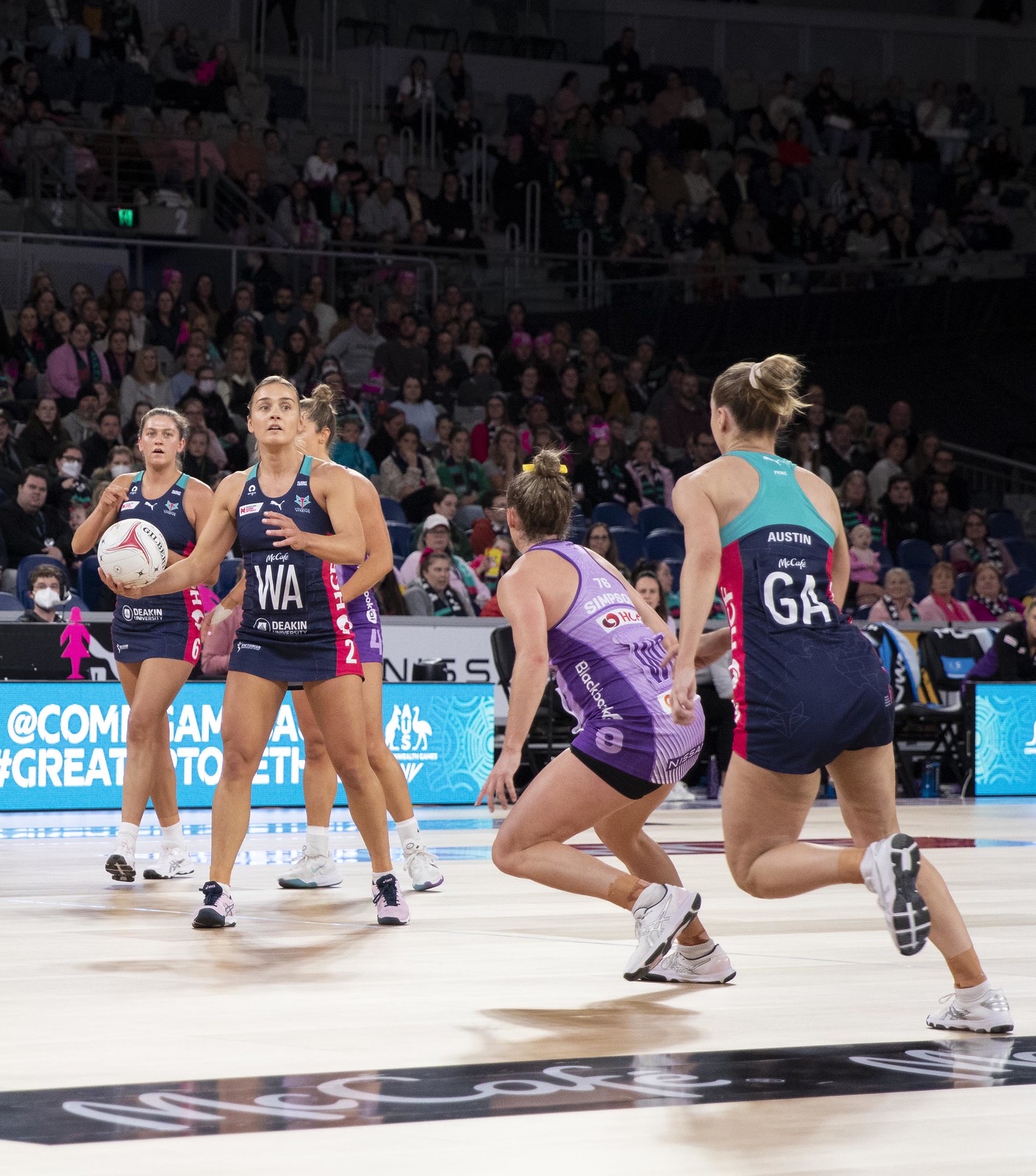The photograph captures an intense moment during an indoor women's sports game inside a gymnasium, evidenced by its polished wooden floor and numerous spectators filling the bleachers in the background. The main focus is on five female athletes engaged in the game. On the left side, a player wearing a navy blue and teal uniform, distinguished by a pink strip along the sides, holds the ball as she prepares for a move. Directly in front of her, a player from the opposing team in a purple uniform appears ready to attempt a steal. Behind the ball-handler, another teammate in navy and teal looks poised to provide support or block the approaching adversary. Further to the right, another pair of athletes—one in navy and teal, and one in purple—are also engaged in the action. The gym's blue and white banners are partially obscured by the players, but a black floor decal prominently features the word "Maccafe," reflecting the vibrant and competitive atmosphere of the ongoing game.